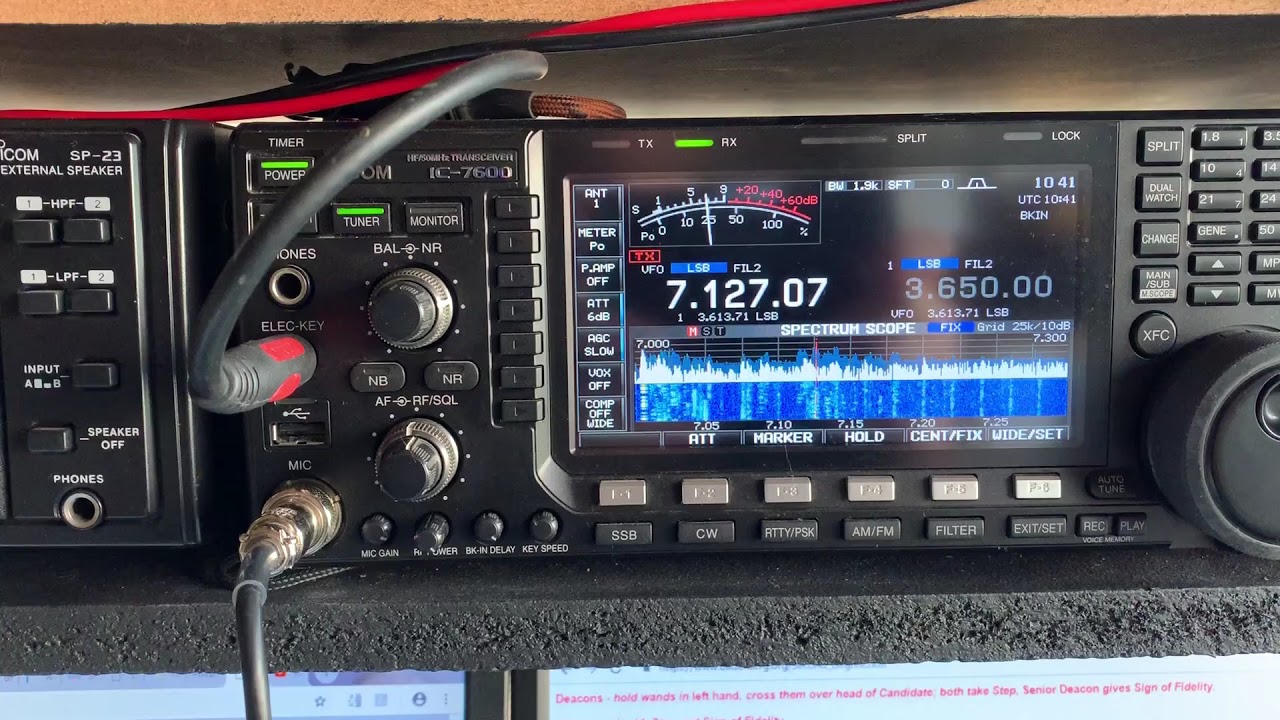The image depicts a detailed close-up of a stereo receiver. Prominently positioned in the center, the receiver features a digital display labeled "Spectrum Scope" with white text. Above the display, numerical readouts on the left and right show "7.127.07" and "3.650.00," respectively. The decibel meter ranges from 0 to 60, with the 20 to 60 section highlighted in red. Below the display, two rows of buttons are visible: the top row comprises gray buttons labeled from "F.2" to "F.6," and the bottom row features black buttons marked "SSB," "CW," "RTTY," "PSK," "AM," "FM," "Filter," and "Exit." Additional smaller buttons nearby read "Auto-Tune," "Record," and "Play." 

Towards the lower right corner of the receiver, there is a large dial, with a keypad positioned above it. To the upper middle of the image, a red and black cord connects to a black auxiliary cord, which extends to the left middle of the image, plugging into the Alec key. Multiple open jacks are present for phones and a microphone, and the mic port has a plug inserted. Dials for balance and equalization flank these sockets. On the left side of the image, additional elements include the speaker, keypad, and another phone jack. The setting appears to be indoors, possibly in a work environment, with a variety of colors visible: blue, light blue, purple, black, gray, silver, lime green, red, and orange.